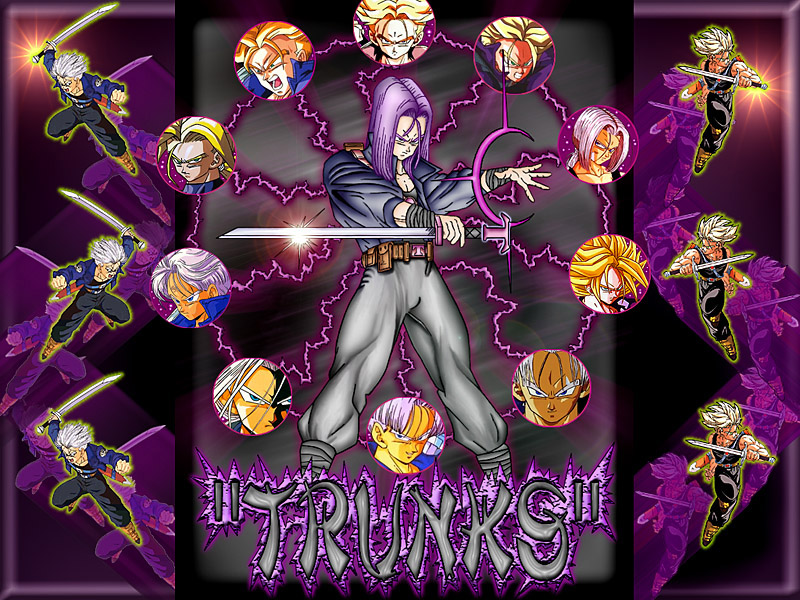This captivating anime artwork features a central figure with long purple hair, clad in a blue shirt, grey trousers, and a brown belt. He stands with his legs apart, brandishing a sword in his right hand and extending his left hand, as if casting a spell. Encircling him are ten round illustrations of various anime characters, each distinctly detailed. The background is a striking gray metallic with stylized elements, including the word "TRUNKS" in elaborate silver script at the bottom. Flanking the central figure are three characters on each side, all wielding knives or swords. Purple squiggly lines connect these characters to central circles, creating an intricate, interwoven design that adds to the dynamic energy of the scene. The overall color palette combines shades of purple, grey, and black, accented with yellow, enhancing the dramatic effect of the illustration.